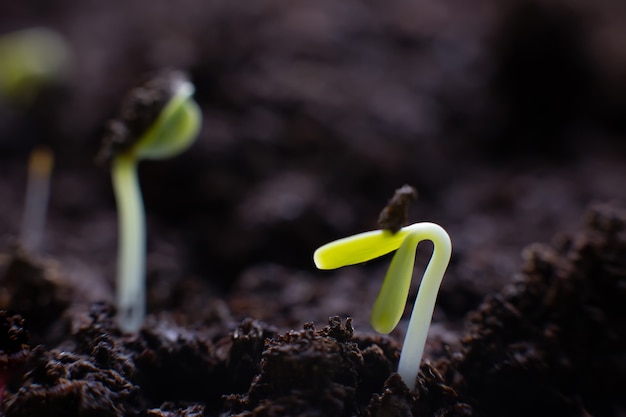In the photograph, presented in a landscape layout with a predominantly dark and very blurry background, the foreground clearly depicts the rich, textured brown soil occupying the bottom 20-25% of the image. Emerging from this soil are several very young and fragile budding plants. Two prominent plants stand out: the first, centrally located with a slight shift to the right, features a thin white stem transitioning to green as it extends upward, before bending over and splitting into a Y-shape with small green pods at its tips. This plant appears to be weighted down by a small clump of soil adhering to its top section. The second plant, positioned more towards the left-hand side, is similarly thin and white, with tiny green protuberances at the top. This plant stands more upright yet still appears delicate. The details of the background are intentionally out of focus, emphasizing the new sprouts' nascent growth amidst the dark, fertile earth. No people or text are present in this serene and intricate image capturing the early stages of life for these plants.